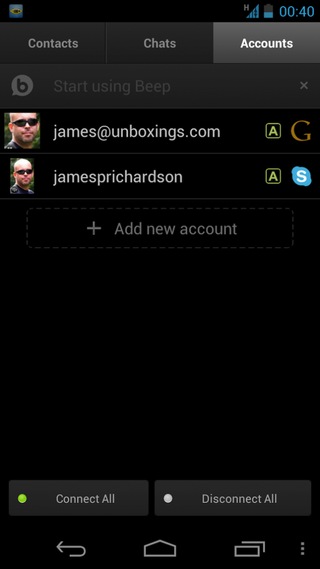The image, captured from a smartphone, features a dark interface with a black background. In the upper right corner, the timestamp reads "00:40," and the battery indicator shows approximately one-third remaining. Below this, the screen is divided into three sections labeled "Contacts," "Chats," and "Accounts," with "Accounts" highlighted in gray with white text.

Beneath this header, text in dark gray on a slightly darker gray background reads "Start using Beep."Centered below this text is a small photograph icon of a white male wearing sunglasses and looking directly at the camera, labeled "James at Unboxing.com." In the upper right corner of this section, the letters "A" and "G" are displayed.

Following that, a similar but slightly larger picture icon of the same individual appears, now showing the top of his bald head. Next to this, the name "James P. Richardson" is displayed along with the letters "A" and "S" to the right.

Further down the screen, there's an option indicated by a plus sign with the text "Add new account." The bottom portion of the screen features a largely empty black space. Towards the very bottom, a dark gray box contains a neon green circle with the text "Connect all." Adjacent to this is another dark gray rectangle with a white circle and the words "Disconnect all."